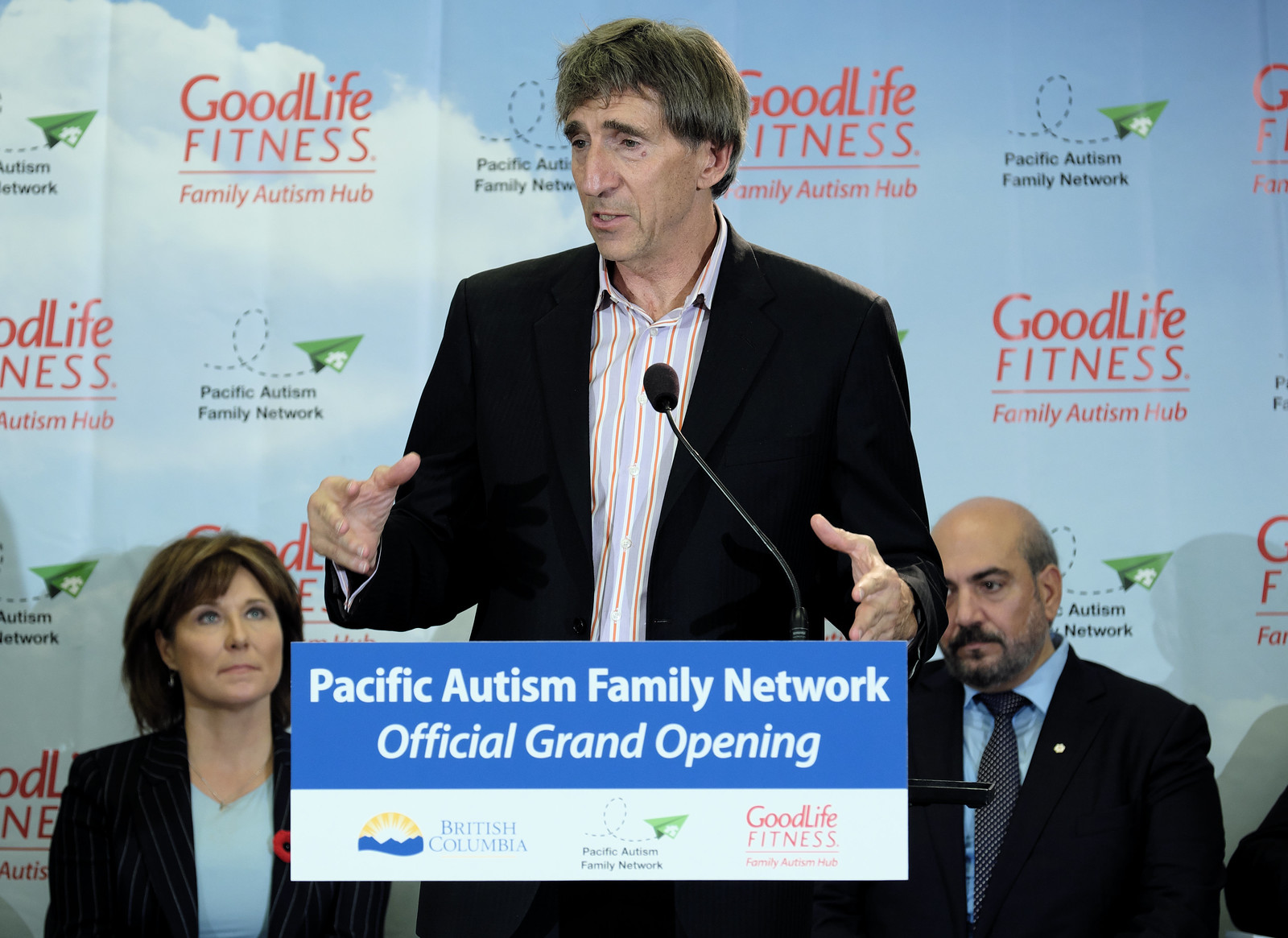This image features a spirited Caucasian man with disheveled brown hair standing at a podium during an event. He is wearing a black suit coat over a gray dress shirt with vertical red stripes and is passionately addressing the audience with his hands gesturing in front of him. Behind him, the backdrop is adorned with logos for Good Life Fitness, Autism Hub, and Pacific Autism Family Network, all set against a blue sky with cloud imagery and a lime green glider making a loop. The podium's sign reads "Pacific Autism Family Network Official Grand Opening," with additional logos for British Columbia and Good Life Fitness displayed below. Seated behind the speaker to his right is a bald man wearing a blue dress shirt, black coat, and tie, who appears rather solemn. To the left is a woman with variegated brown hair with streaks, wearing a pinstripe jacket over a pale blue shirt, attentively looking at the speaker. This Canadian event, dedicated to autism and family healthcare, showcases a collaboration among several organizations working together for autism solutions.